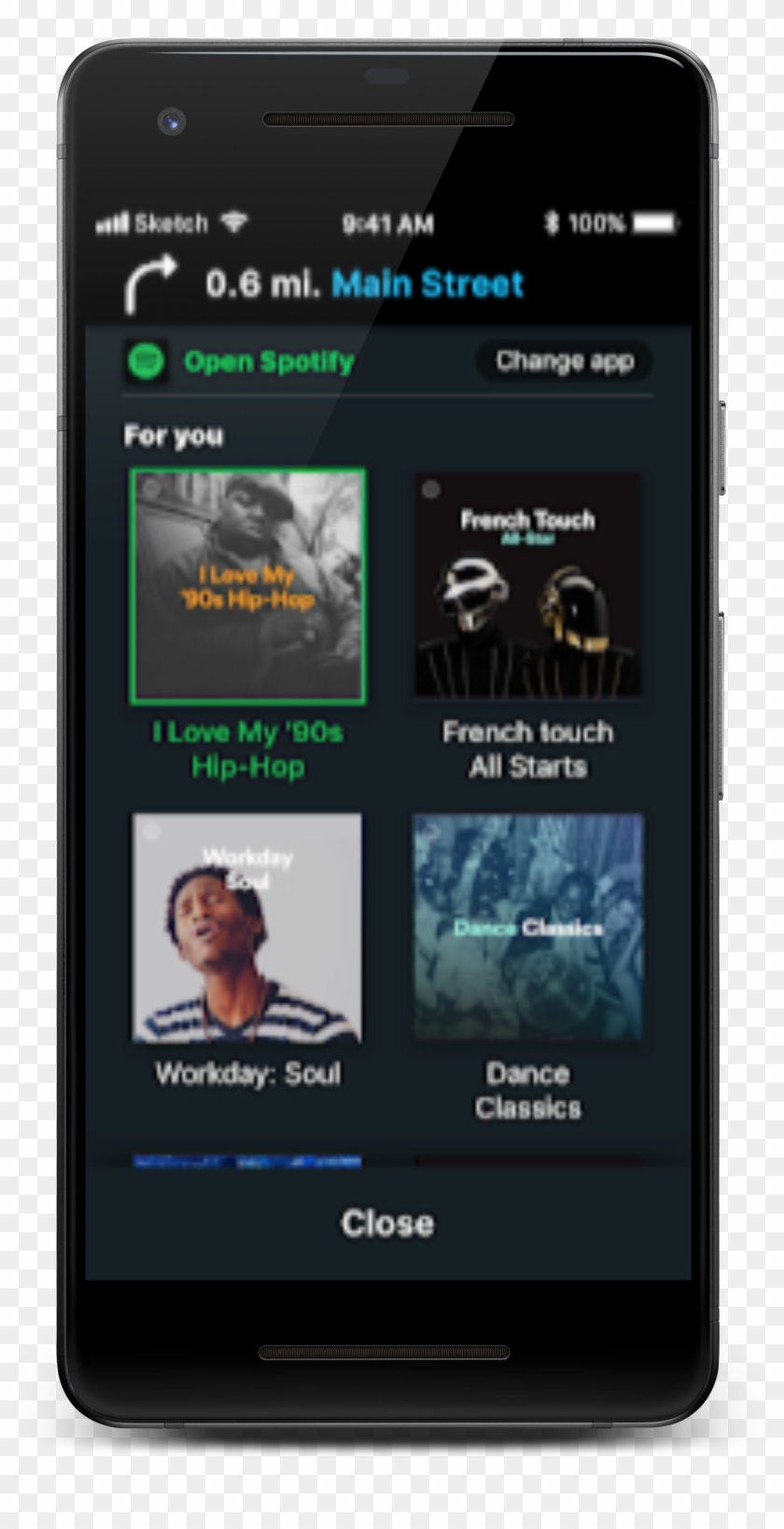This detailed caption could accompany the image described:

"In this screenshot of a mobile device with a predominantly black background, two main elements are displayed. At the very top, a navigation interface provides driving directions, indicating an upcoming right-hand turn in 0.6 miles onto Main Street. Positioned beneath the navigation bar is a Spotify playlist featuring four distinct albums. The albums listed are: 'I Love My Nineties,' 'French Touch,' 'Workday Soul,' and 'Dance Classics.'"